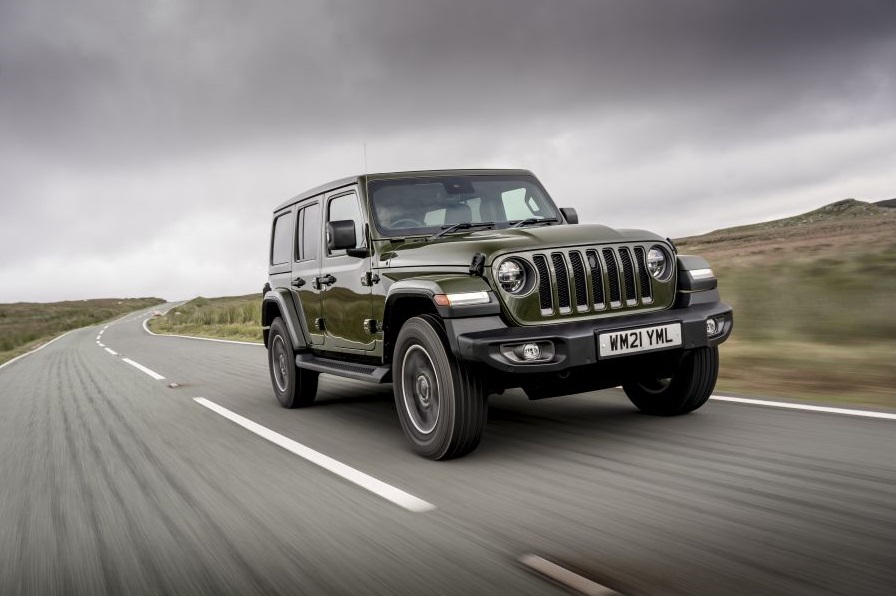The image captures a dynamic scene of a modern, right-hand drive, dark green Jeep Wrangler, potentially a 2023 or 2024 model, driving down an empty two-lane asphalt road with white center lines. The Jeep, sporting a white front license plate reading "WM21 YML", is equipped with distinctive features like four doors, round headlights paired with a vertical grill, hood latches, black plastic fender flares, and a side step. The motion is evident as the tires spin and the surrounding road and fields blur, emphasizing the vehicle in action. The backdrop paints a serene, yet dramatic picture of a meadow-like environment with knee-high grasses stretching into the distance, accompanied by rolling hills and an overcast sky, filled with dark clouds hinting at impending rain.